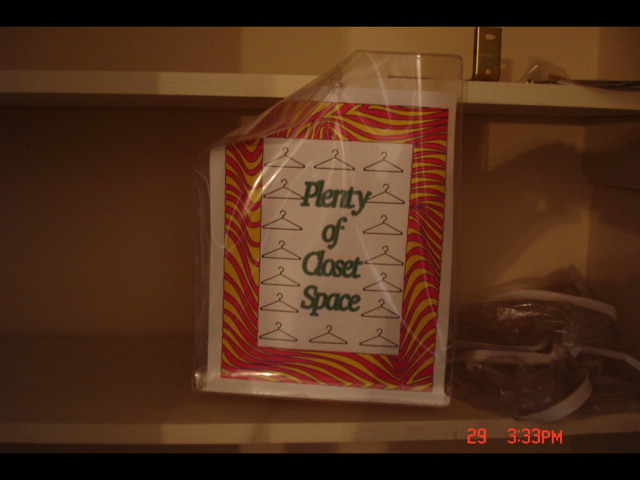The photograph depicts a dimly lit, indoor scene focused on a set of fiberboard shelves with a light wood grain finish. Centrally tacked onto one of the shelves is a printed piece of paper protected by a plastic cover. The paper is adorned with a red and gold floral border, and in the middle, bold green text reads "Plenty of Closet Space," surrounded by illustrations of black coat hangers. To the right of this sign, there is a pile of plastic bags with zippers, likely used for storing garments or shoes. The image captures the shelves fairly empty, emphasizing the sign and storage bags. A time stamp in red, "29 3:33 p.m.," is visible in the bottom right-hand corner, adding temporal context to the scene. The soft lighting and shadow cast by the photographer add a subtle depth to the overall composition.